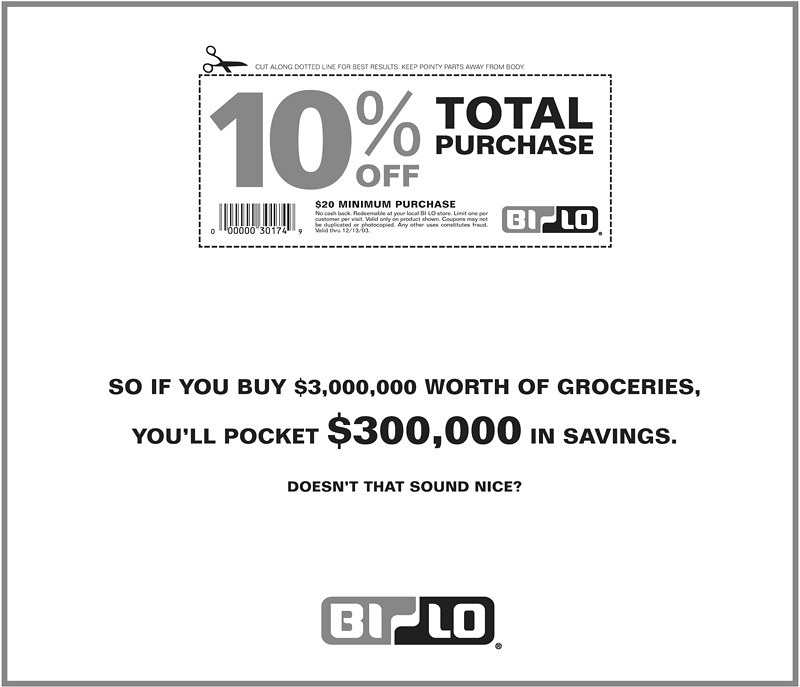This black-and-white advertisement for Bilo features a medium gray border encasing the entire image. Prominently displayed at the top is a detailed coupon, highlighted by a black scissors icon and a dotted line urging, "Cut along dotted line for best results, keep pointed edges away from body." The coupon offers "10% off total purchase" in a mix of gray and black text, with a stipulation of a $20 minimum purchase. A barcode labeled "00000030174" is situated on the bottom left of the coupon, accompanied by small text that includes "no cash back, redeemable at your local Bilo store, limit 1 per customer," although this text is somewhat difficult to read. The Bilo logo, which resembles two puzzle pieces about to snap together, appears at the bottom right of the coupon. Directly below the coupon, in a bold and whimsical font, the ad humorously states, "So if you buy $3,000,000 worth of groceries, you'll pocket $300,000 in savings. Doesn't that sound nice?" The validity period of the coupon, which expired on December 13th, 2003, is subtly included, adding a touch of nostalgia. At the very bottom center of the ad, the Bilo logo is reiterated, grounding the entire advertisement in its branding.